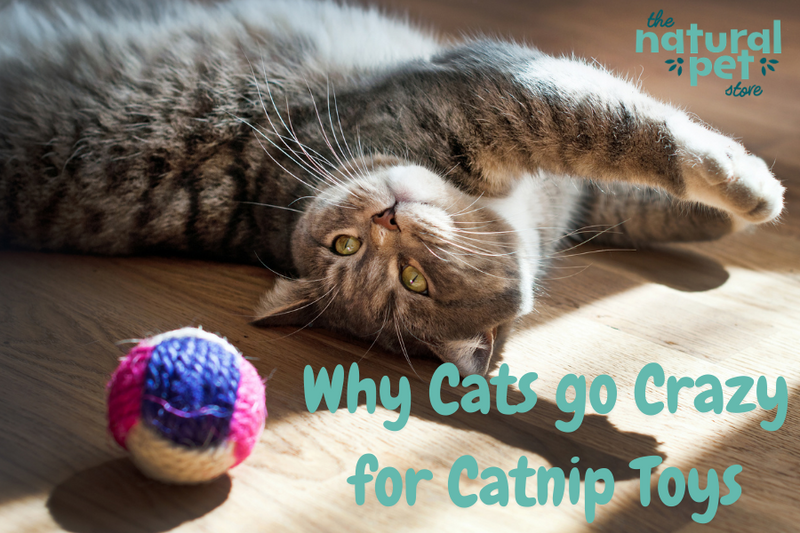This indoor photograph captures a gray tabby cat lounging on a brown wooden planked floor. The cat is positioned towards the upper left-hand corner, stretched out on its back with its white-tipped paws extended forward, and its white chest and mouth accentuating its gray-striped fur. The cat's head rests on the floor with greenish-yellow eyes gazing up towards the left, partially illuminated by a beam of sunlight that casts a gentle shadow. In the upper right-hand corner, the text "The Natural Pet Store" is prominently displayed in blue. A colorful yarn ball, woven from white, blue, and pink strands, sits in the lower left-hand corner. Beneath this, in large blue print, the words "Why Cats Go Crazy for Catnip Toys" highlight the playful scene, suggesting the image could be part of an advertisement for The Natural Pet Store, emphasizing the joy cats find in catnip toys.